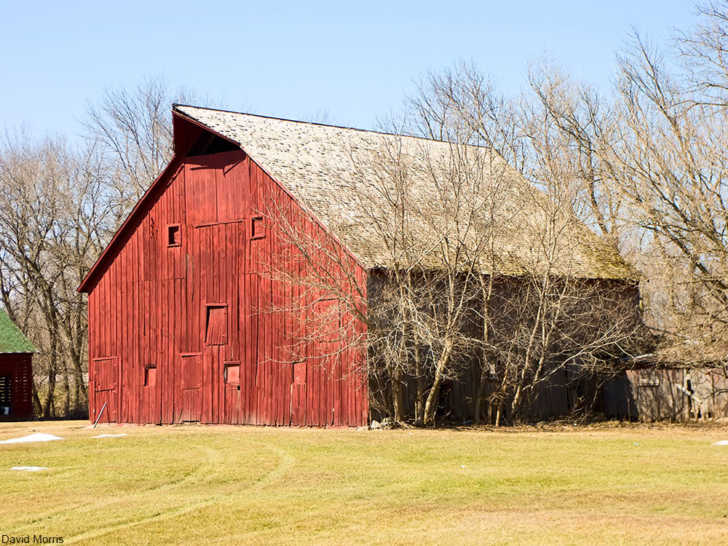This image showcases a realistic-looking, horizontally framed photograph of an old red barn under a bright, clear blue sky. The barn, with its traditional two-story structure, features a large, slanted light gray roof and several shuttered windows and doors, all painted the same bright red as the wooden exterior. The windows appear to be covered, and there is a prominent black text that reads "David Morris" in the bottom left corner.

Surrounding the scene are tall, leafless trees, indicating a late fall or winter season. The grass in the foreground is a mix of light green and brown, with visible tire tracks leading up to the barn. There is a wooden fence flanking both sides of the barn, with some planks missing. 

To the left of the main barn, partially cut off in the image, is a smaller red shed with a green roof. The sky above is a cloudless, vivid blue, adding to the overall tranquil yet slightly weathered ambiance of this rustic rural setting.